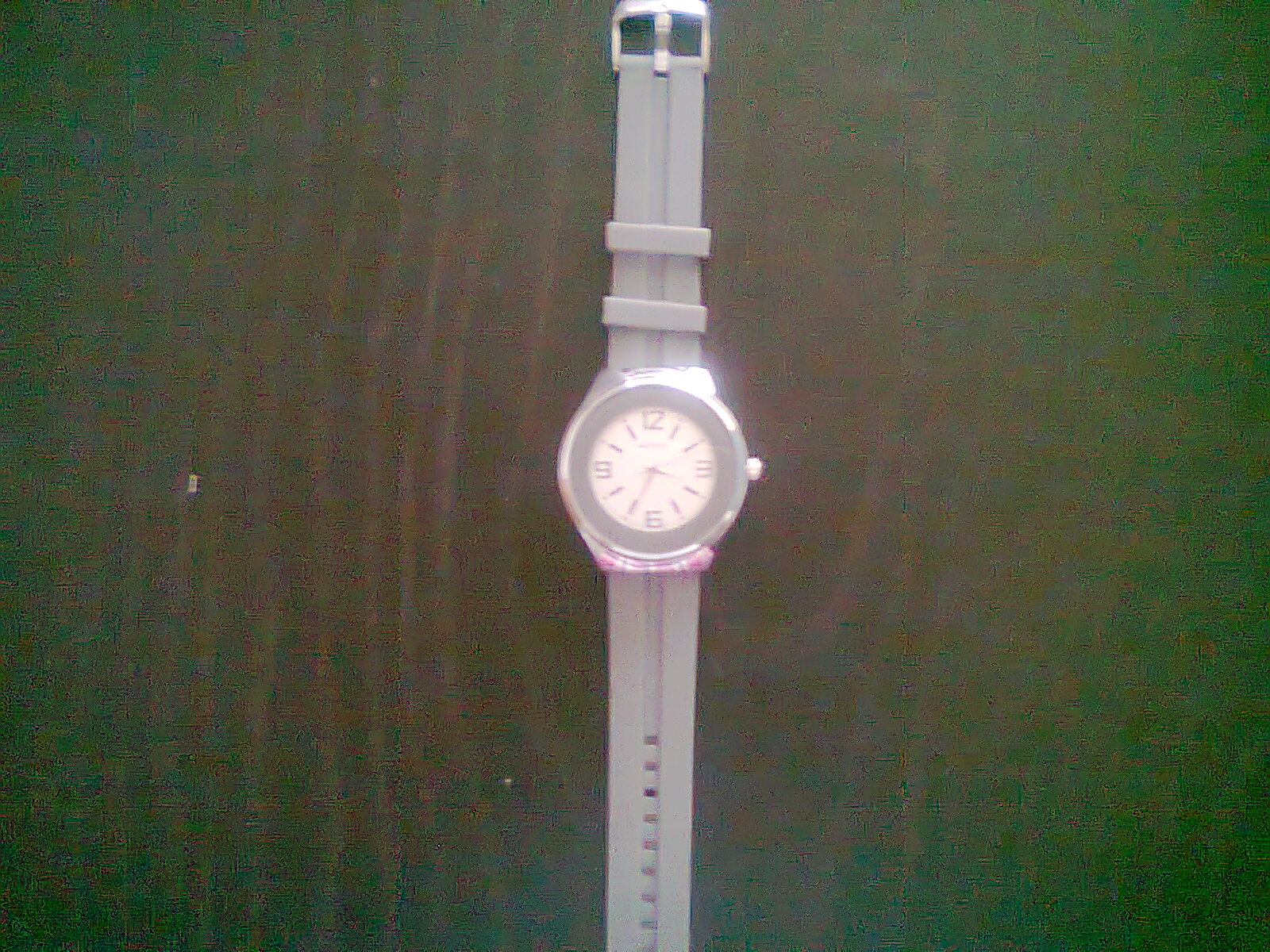This color photograph captures a close-up view of a wristwatch placed on a dark wooden surface. The watch, centered in the image, features a gray rubber band with the metal buckle extending slightly beyond the top edge of the frame. Despite the blurriness of the photo, one can discern the watch's white face adorned with black numerals marking the 12, 3, 6, and 9 o'clock positions. The remaining hours are indicated by thin black vertical lines. The watch hands, also black, stand out against the white background. A winding knob is visible on the right side of the watch case. The image does not contain any writing, people, or animals.